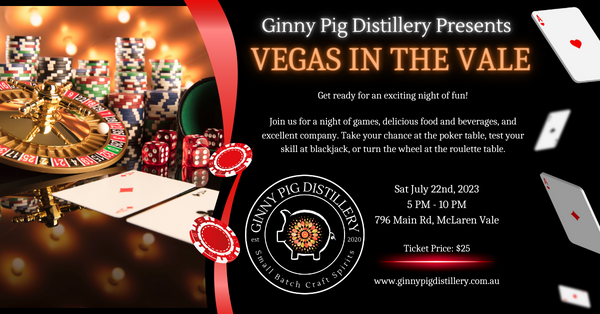This advertisement for an event at the Guinea Pig Distillery features a long, rectangular design with a black background. On the left side, there's a vivid image showcasing a roulette wheel, stacks of poker chips, two white-backed playing cards, and red dice laid out on a shiny black table, illustrating a classic casino night ambiance. A vertical red ribbon with the graphic of two poker chips divides the left image from the right side of the advertisement. To the right, the black background continues prominently, featuring the white text, "Guinea Pig Distillery Presents," followed by the event title "Vegas in the Veil" in bold gold letters. Below this, a detailed description invites guests to enjoy a night of games, delicious food, beverages, and excellent company, with specific highlights like poker, blackjack, and roulette. The event takes place on Saturday, July 22, 2023, from 5 p.m. to 10 p.m. at 796 Main Street, McLaurin Vale, with a ticket price of $25. Additionally, the rightmost edge of the advertisement is bordered with floating playing cards, and a large circular Guinea Pig Distillery logo is prominently displayed in the middle of the right section.